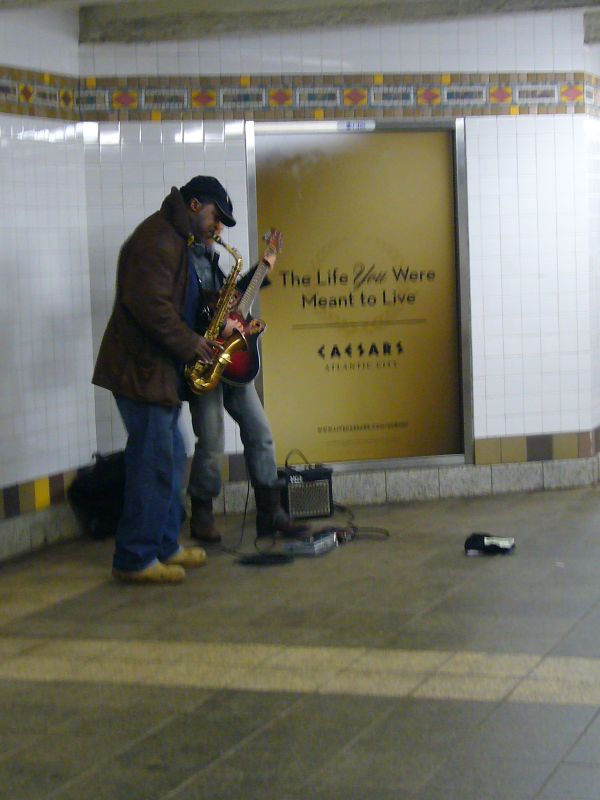In an underground train station, two men are performing music in front of a white-tiled wall with a gray and yellow border featuring hints of red and orange. One man, dressed in jeans, a brown jacket, and a baseball cap, is playing a polished electric guitar connected to an amplifier. The other man, clad in a blue coat, jeans, and boots, is playing a brass saxophone. Both musicians appear to be busking, with a hat placed on the grayish-brown tile floor likely to collect tips, surrounded by their speakers and bags. Behind them, a prominent yellow sign with black writing reads, "The Life You Were Meant to Live, Caesars," suggesting an advertisement for Caesars Casino. The setting is also detailed with a line of lighter-colored tiles that runs down the center of the walkway, enhancing the depth and context of the scene.